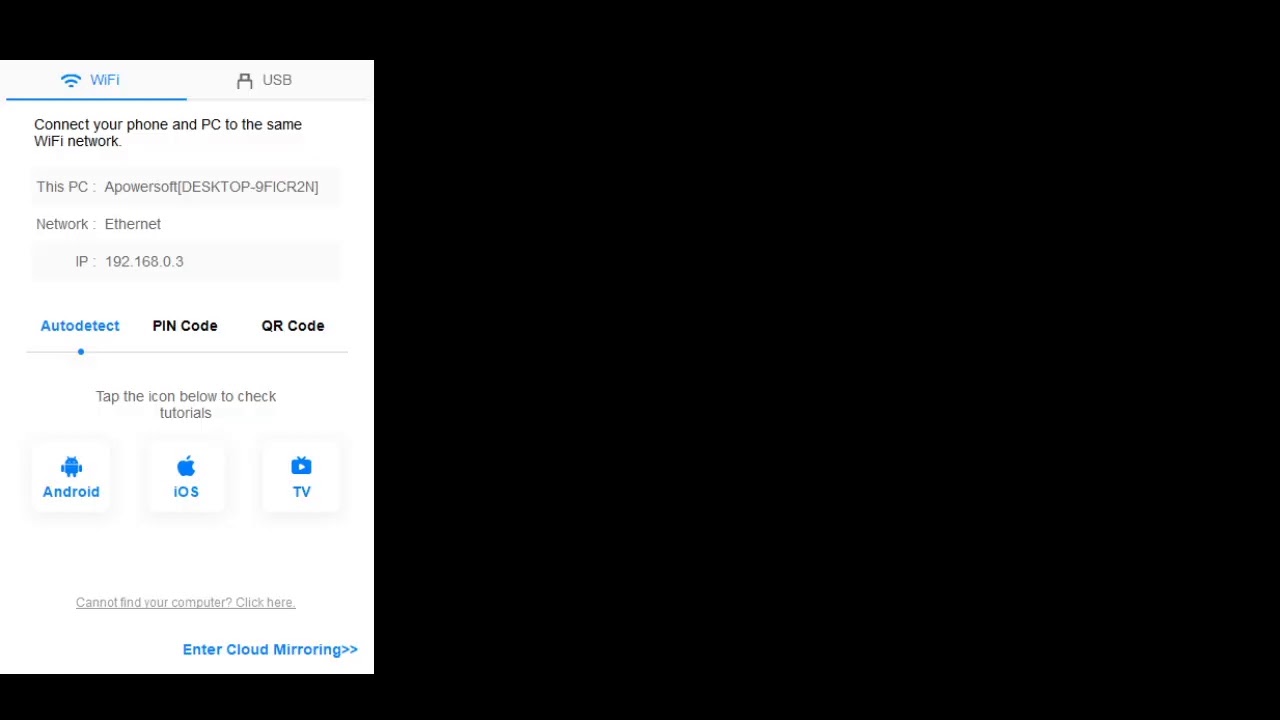The image features a predominantly black background on the left side. On the right side, there is a detailed screenshot from a phone, displayed against a white background. At the top of the screenshot, a blue Wi-Fi symbol is shown next to the word "Wi-Fi." To the right of this, the term "USB" is displayed in black alongside its corresponding symbol.

Below this, the text instructs users to "Connect your phone and PC to the same Wi-Fi network." Following this, the screenshot provides specific details about the computer connection, reading "This PC: ApowerSoft (DESKTOP-9F1CR2N), Network: Ethernet, IP: 192.168.0.3."

Further down, the options for "Auto Detect," "Pen Code," and "QR Code" are listed, followed by the instruction "Tap the icon below to check tutorials." Three boxes are presented underneath, each containing a different symbol and label: "Android" with the Android logo, "iOS" with the iOS logo, and "TV" with a TV icon.

At the bottom, there is a message stating, "Cannot find your computer? Click here," written in blue. Just below this, also in blue, the text reads "Enter Cloud Mirroring" accompanied by an arrow symbol pointing to the right.